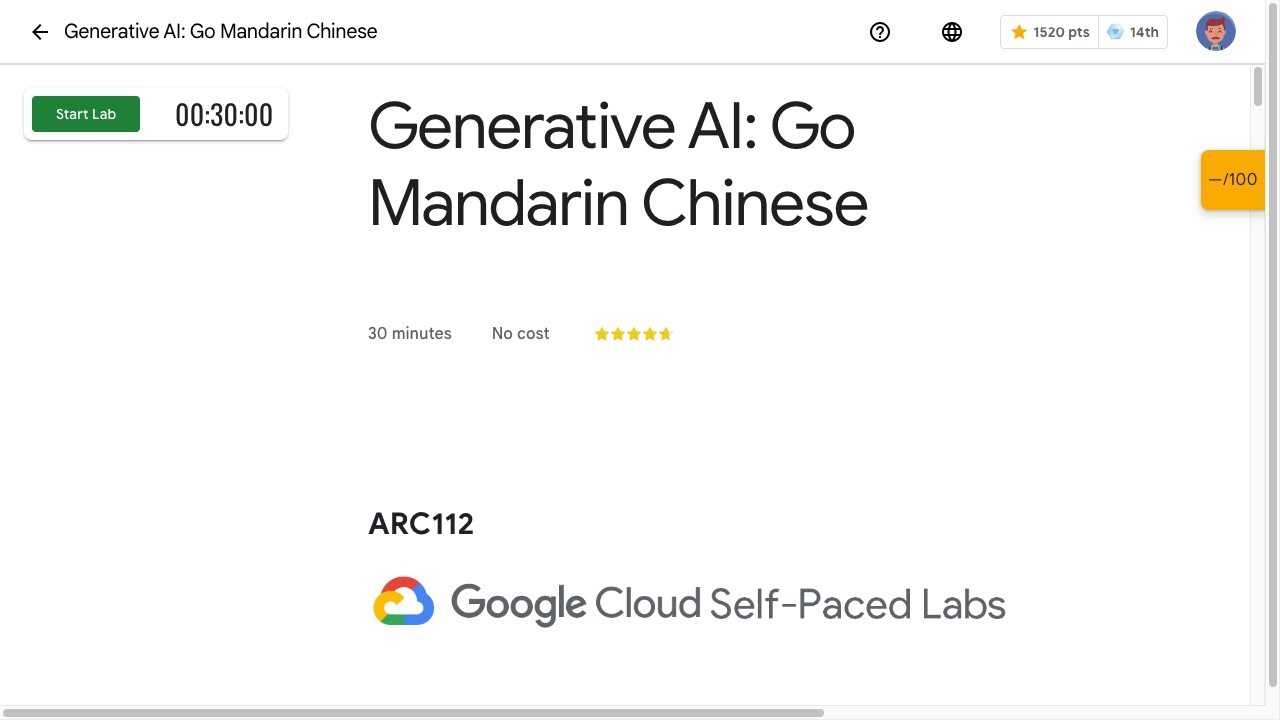In the upper portion of the image, a black arrow points to the left. Beside it, the text "Generative AI... Go Mandarin Chinese" is displayed in black font. Below this, a white circle outlined in black contains a black question mark. Adjacent to the circle, there's a grid design with intersecting horizontal and vertical black lines. 

Further down, there's a white rectangle with a gray outline featuring a yellow star and the text "1520 points". Next to this, a blue hexagon indicates "14th", and within the hexagon, there is a circular image of a light brown-haired animated character set against a blue background. A gray line extends horizontally across the section, with the text "Generative AI... Go Mandarin Chinese" repeated below it in black font.

On the right side, an orange square contains black text with a dash, a slash, and the number "100", which might signify a score. The text "30 minutes no cost" is also displayed in black font, followed by a near five-star rating, with just the tip of the last star not filled in yellow.

Towards the bottom, there is some spacing before the bold, capitalized text "ARC 112". Underneath, a logo resembling Google Cloud is placed, with the text "Google Cloud Self-Paced Labs" in gray, where each word begins with an uppercase letter.